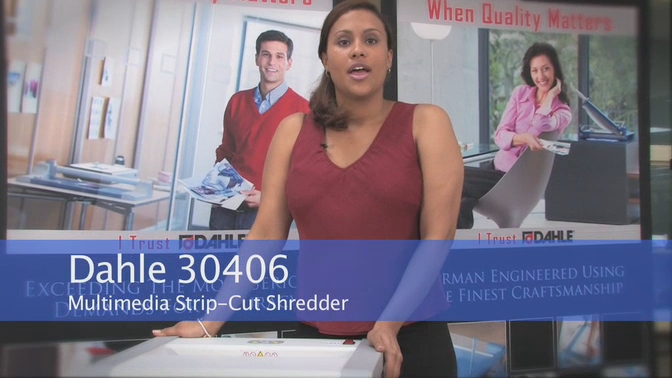The image is an advertisement for the "DAHLE 30406 Multimedia Strip Cut Shredder," showcasing a product engineered with the finest German craftsmanship. At the center of the photo stands a woman, potentially Hispanic or mixed race, with brown hair pulled into a side ponytail. She is wearing a red tank top and black pants, and she rests her hands on the shredder. The text around her reads, "Multimedia Strip-Cut Shredder, engineered using the finest craftsmanship," and "I trust DAHLE."

Flanking the central figure are two smaller images set in office environments. On the left is a man in a red sweater over a blue button-down shirt, holding a piece of paper with paneled walls behind him adorned with paper. On the right, there is an Asian woman in a pink shirt, sitting in a chair in what appears to be an office. In the forefront, a blue strip prominently displays "DAHLE 30406 Multimedia Strip Cut Shredder." The backdrop includes slogans such as "When Quality Matters," emphasizing the product's superior build.